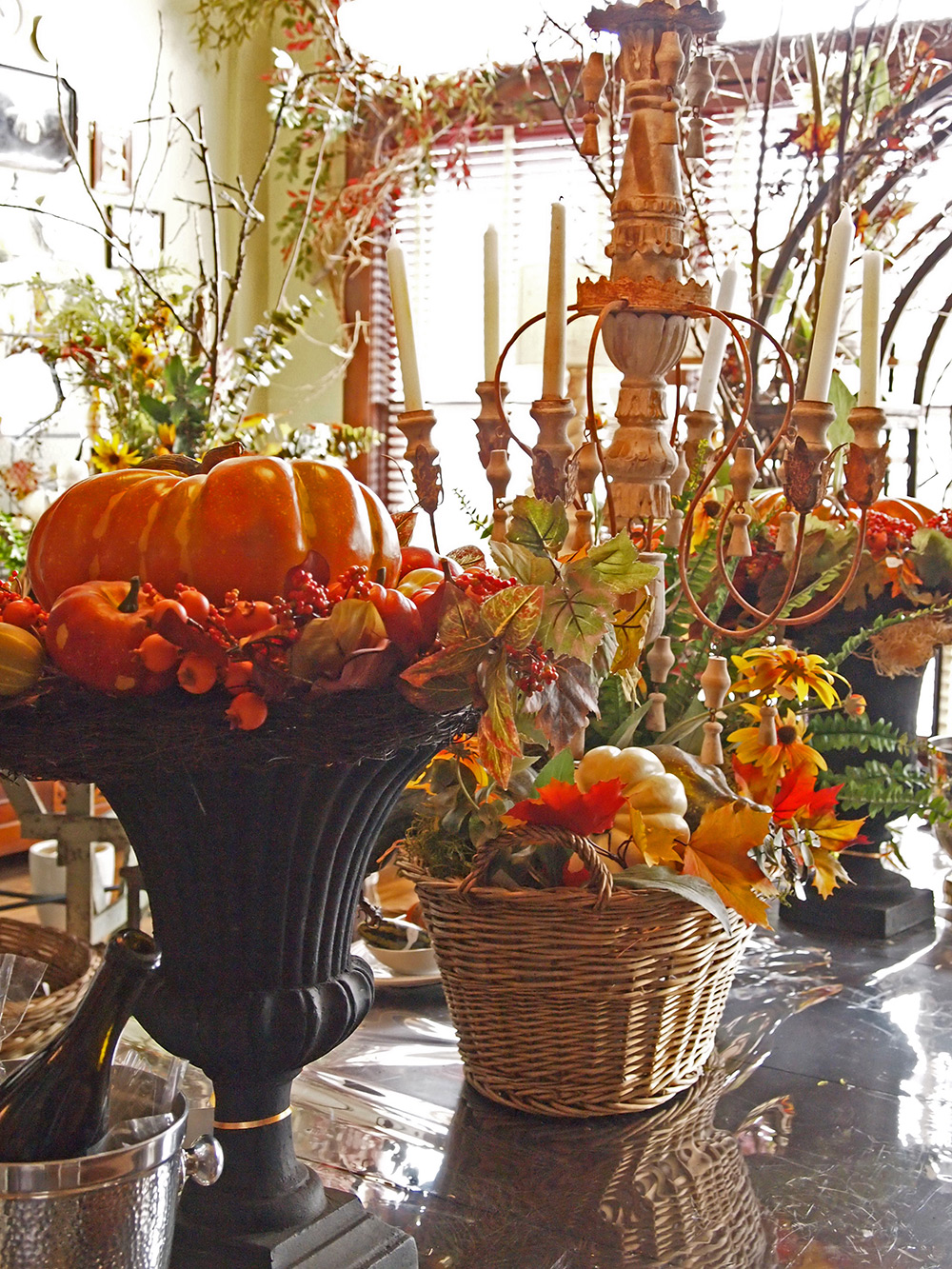This photograph captures a detailed autumn-themed display atop a black table. In the bottom left corner is a silver bucket holding an open wine bottle. To the right of the bucket is a striking black urn vase containing a large orange pumpkin, surrounded by smaller pumpkins and various other fruits and vegetables. Centrally positioned is a brown wicker basket overflowing with white pumpkins and orange-hued dried flowers. Just behind this basket stands a tall candelabra adorned with six unlit white candles, each set in a golden tan, brown, and white holder. The background features a brightly lit window with partially open blinds allowing sunlight to filter through. Additional elements include some visible tree branches, greenery, and flowers peeking from behind the arrangements, as well as picture frames mounted on the wall in the upper left section of the image. The gray floor contrasts with the rich autumnal colors and textures of the display, creating a cohesive and inviting scene that epitomizes fall decor.